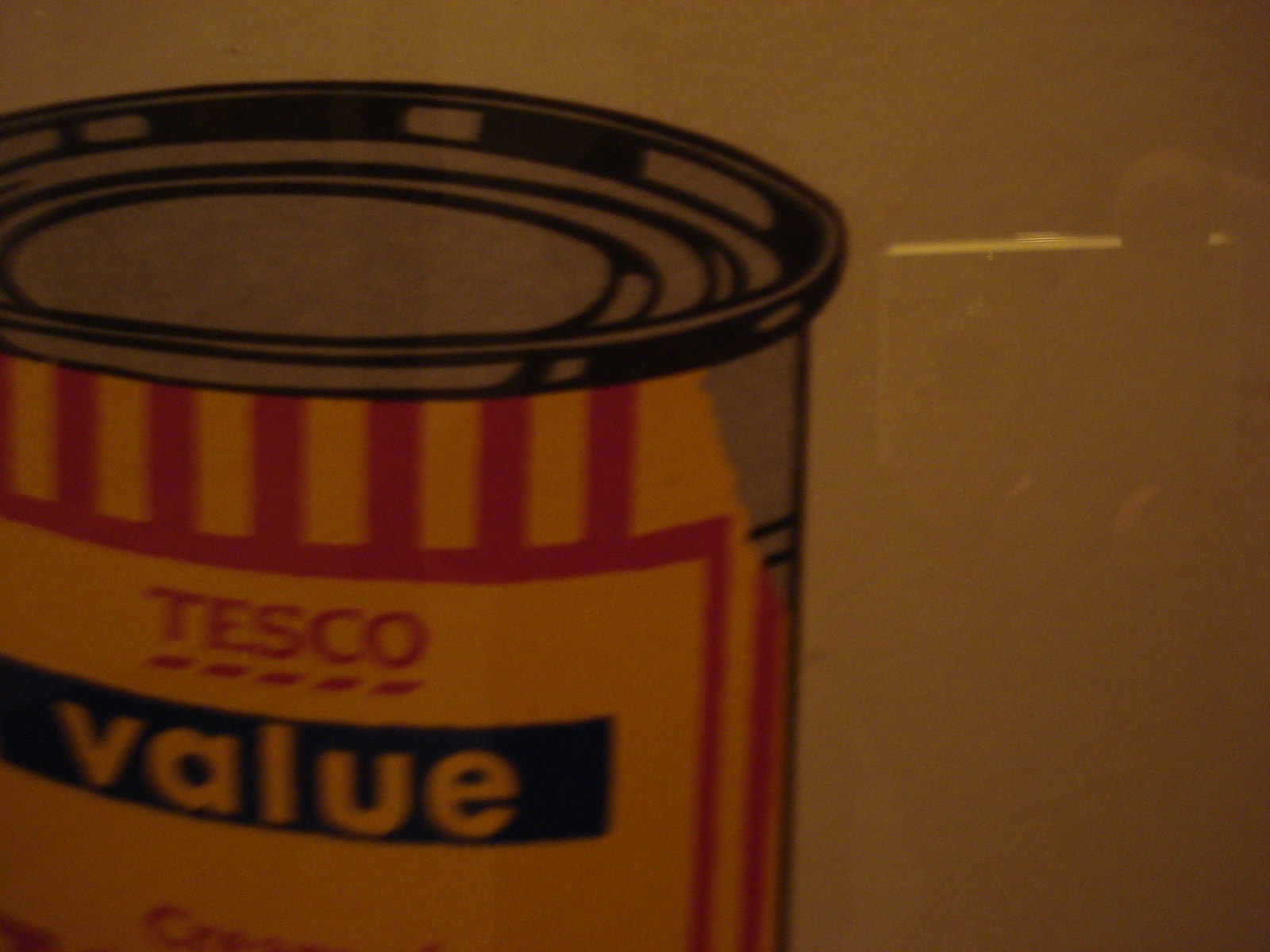This detailed caption describes a vintage Tesco aluminum can, depicted in an artistic drawing. On the right side of the image, a person's hand is visible, holding a phone and capturing a photo of the drawing. The left side showcases the old, partially ripped label of the Tesco can, with significant portions missing on the right side. The can appears predominantly white, featuring a red square enclosing six small red rectangles arranged at the top. Within this red square, the word "Tesco" (spelled T-E-S-C-O) is prominently drawn, underscored by red lines. Below this, the word "Value" (spelled V-A-L-U-E) is displayed in white within a blue rectangle. The bottom part of the can is not included in the picture, giving it an incomplete view.